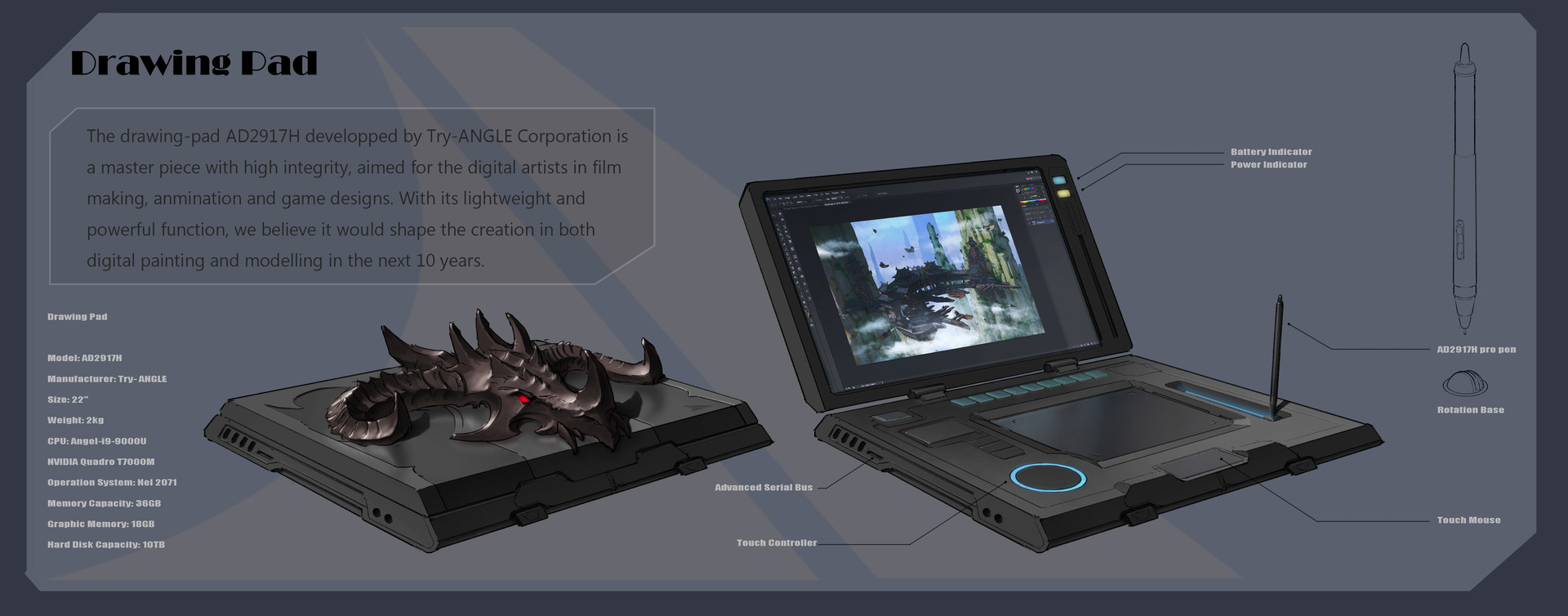The advertisement image depicts a sophisticated digital drawing pad, the AD 2917H, developed by Triangle Corporation. The background and border of the image are grey, with the title "Drawing Pad" prominently displayed at the top in black text. Below, the text reads: "The Drawing Pad AD 2917H, developed by Triangle Corporation, is a masterpiece with high integrity, aimed for digital artists in film making, animation, and game design. With its lightweight and powerful function, we believe it will shape the creation in both digital painting and modeling in the next 10 years." The drawing pad features two screens and can be folded down or up like a laptop. An image on the pad shows a dragon or monster-like character. Additionally, the image highlights various parts of the drawing pad, including arrows pointing to different features, and displays the pen used for inking. The ad's overall grey aesthetics, combined with technical errors in text visibility, contribute to the intricate and somewhat elusive presentation of this high-tech device.